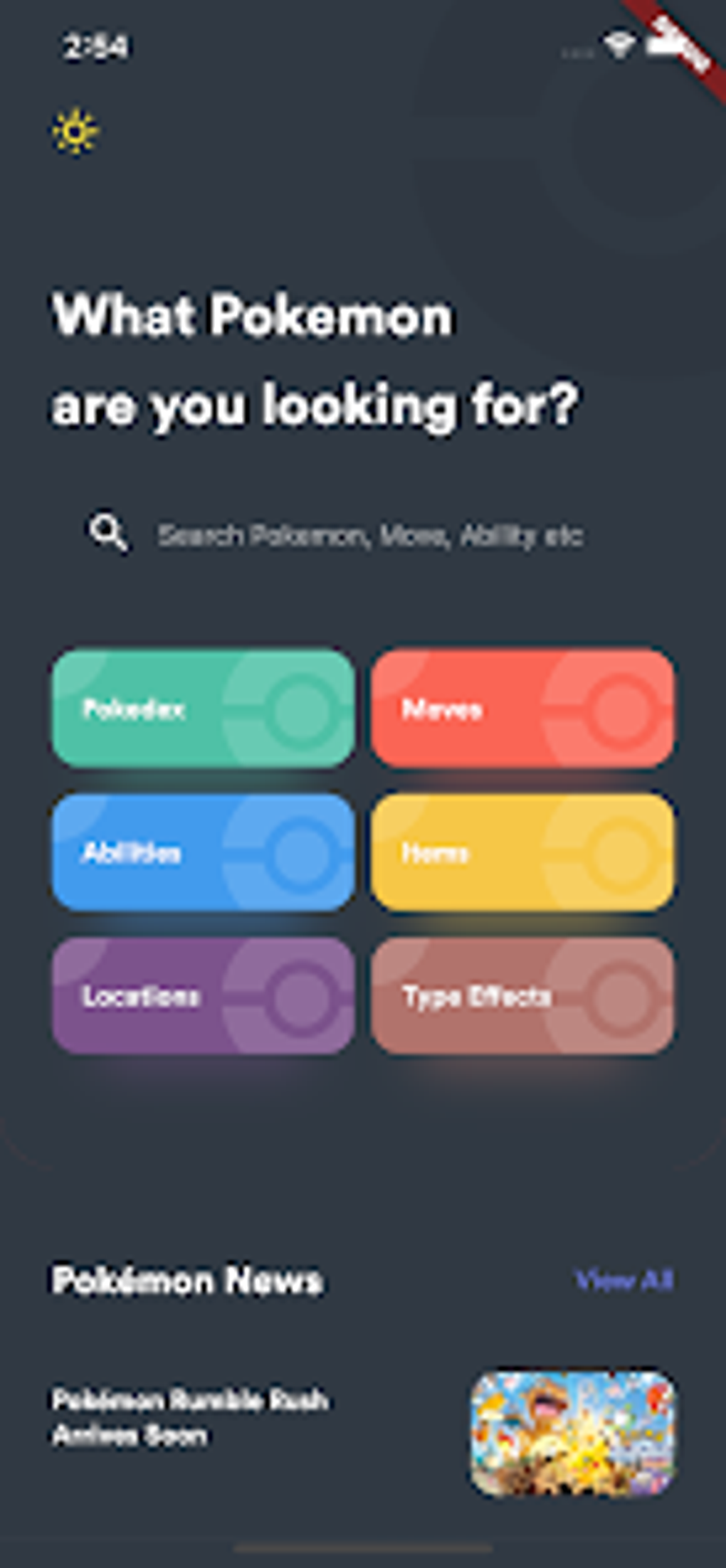The image is a low-quality mobile screen capture with a dark gray background and white text. The top of the screen shows a time of 2:54, accompanied by typical smartphone status indicators: signal strength, Wi-Fi connectivity, and battery life on the top right. On the left, there is a simple sun icon—a yellow circle with radiating lines—indicating daylight.

The main content of the screen features a prompt that reads, "What Pokémon are you looking for?" Below this prompt is a search bar with the placeholder text: "Search Pokémon, moves, abilities, etc." Beneath the search bar, a menu displays several options. Each option has a distinct background color and a white Pokéball icon:
- "Pokédex" with a green background
- "Moves" with a red background
- "Abilities" with a blue background
- An unclear item on a yellow background
- "Locations" on a purple background
- "Type Effects" on a brown background

Below the menu, there is a header titled "Pokémon News" with a clickable link labeled "View All." An article is partially visible underneath this header, but the text is too blurry to distinguish.